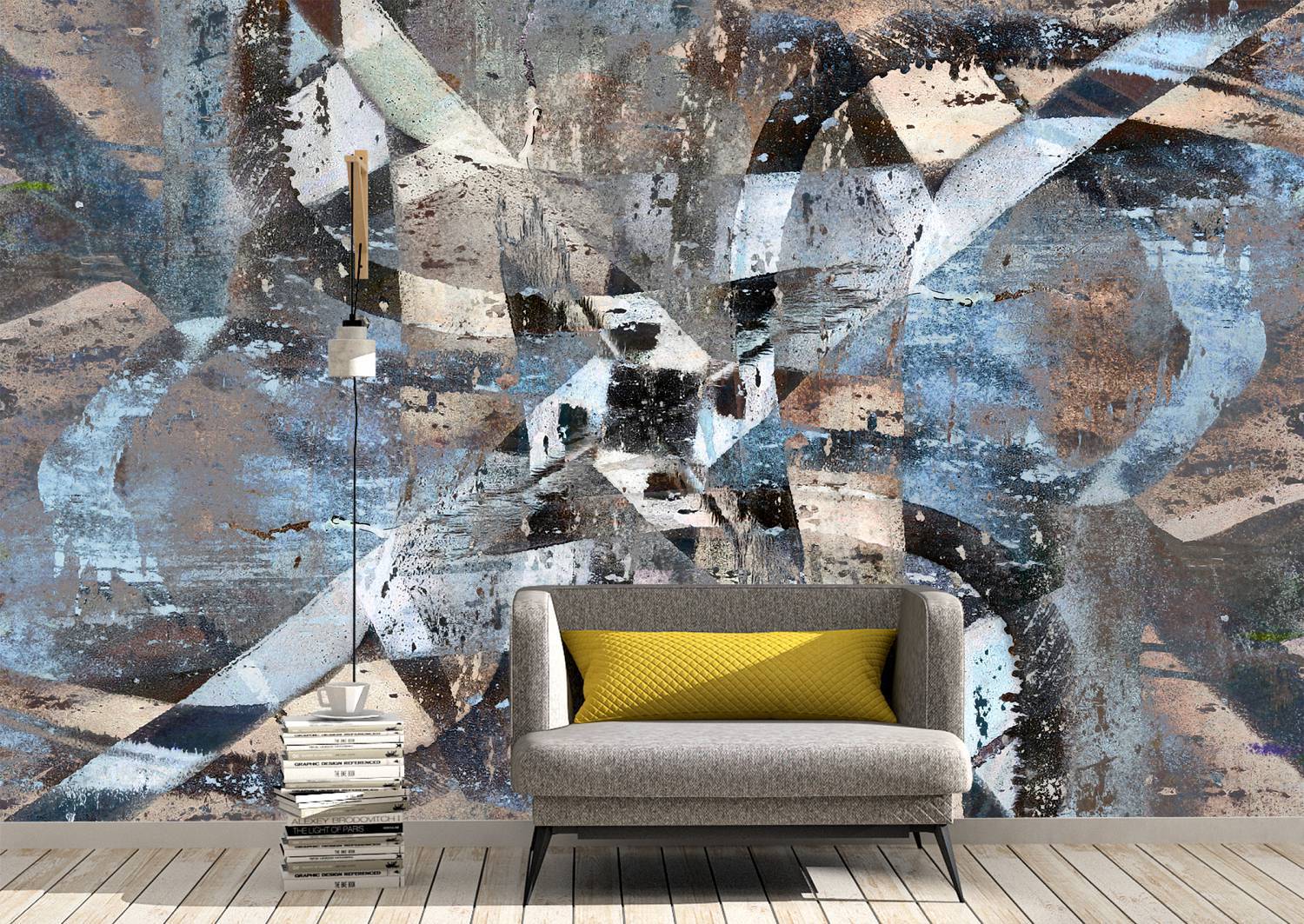In this beautifully designed loft, modern aesthetics meet coastal charm. The interior features striking white wooden floors reminiscent of a beach boardwalk. At the forefront, a sleek gray loveseat with thin, minimalist legs is adorned with a single, vibrant yellow pillow that spans its width, providing a touch of warmth and color. Resting beside the loveseat is an eclectic stack of books with a delicate white teacup perched on top, adding a casual yet sophisticated touch. Adjacent to the seat is an elegantly designed modern pole lamp, characterized by its long, slender frame and a small, pristine white light that dangles gracefully. 

Dominating the backdrop, a stunning wall showcases an abstract mural in swirls of blue, black, and gray, evoking the raw energy and tumultuous beauty of an ocean storm. This artistic feature not only serves as a captivating focal point but also harmonizes with the beach-like ambiance established by the flooring. The overall composition of the room captures a perfect blend of modern functionality and artistic flair, making it both inviting and visually dynamic.